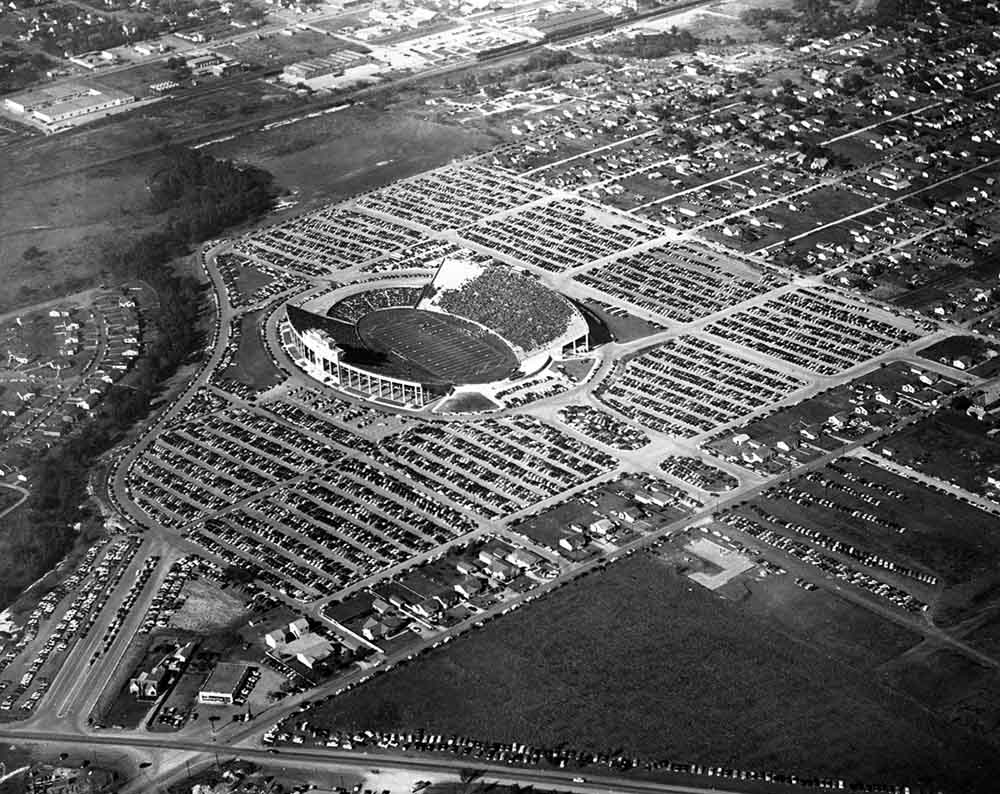A detailed black and white aerial photograph captures a bustling football stadium, characterized by its oval, horseshoe-like open structure with inclining bleachers packed with spectators. The well-attended event is evidenced by the numerous cars filling the surrounding parking lots, suggesting a full house. The picture, seemingly taken from an airplane at an altitude of about 10,000 feet, displays a vast expanse, including a network of highways that stretches horizontally across the lower section, with offshoots leading toward the stadium. To the left and center, rows of trees demarcate the boundary between the parking areas and residential neighborhoods, while similar housing is visible in the upper right corner. The upper left side reveals a mix of white commercial buildings and fields, adding to the urban tapestry around the stadium. The image, likely an old photograph reflected by its black and white nature, captures the significance and centrality of the stadium to the local economy and community.